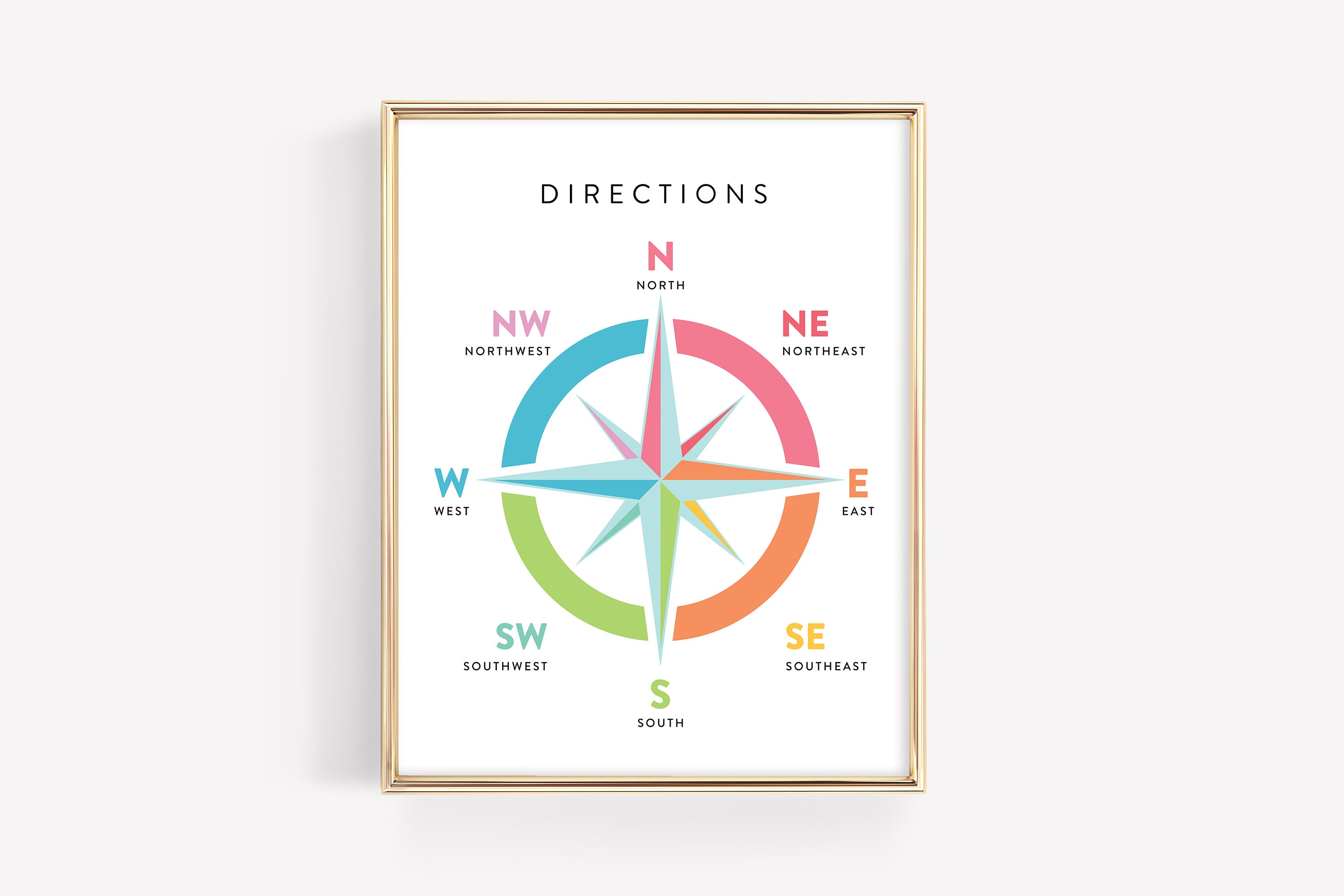Hanging on a blank, white wall, this art print features a gold-framed poster with a centrally-placed compass design. The top of the picture displays the word "DIRECTIONS" in bold, black capital letters. Below this, a compass is centered within a circle that is divided into four quadrants, each distinguished by its own color: pink, orange, green, and blue. The cardinal and intercardinal directions are labeled around the compass in their respective color-coded sections: North (N) and Northeast (NE) are in pink, East (E) is in orange, Southeast (SE) is in yellow, South (S) is in green, Southwest (SW) and West (W) are in blue, and Northwest (NW) is in purple. This vibrant and well-organized print would be perfect for a hiking enthusiast's decor.